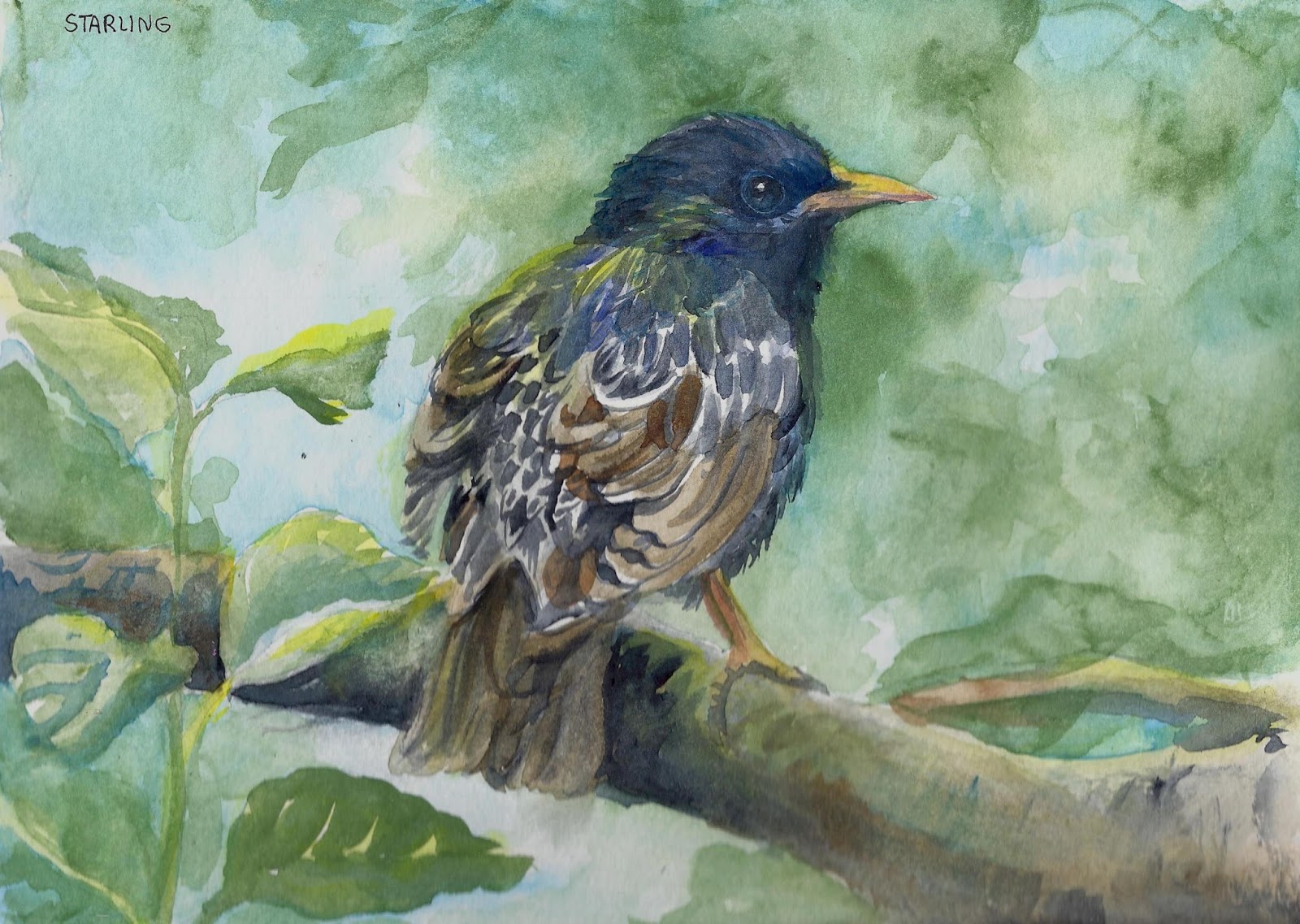This detailed watercolor painting depicts a bird, labeled "Starling" in the upper left corner, perched on a tree limb. The bird, facing right, showcases a striking blend of colors: its smallish yellow beak is long and narrow, and the blue feathers on its head and body mix with shades of navy, medium blue, light browns, tans, and a touch of white to create a delicate feather effect. The bird's tail feathers are dark brown and extend over the limb, which is white on top with a dark shadow beneath the bird and brown on the underside.

The background presents a forest-like scenery, rendered in muted, watercolor shades of green, light blue, and white, giving an impression of light filtering through the canopy. A tall green stalk with broad leaves rises prominently in the foreground, contrasting with the other smudged green leaves painted more abstractly in the background. The small bird's webbed feet clutch the brown log firmly, blending harmoniously with the intricate and vivid surroundings.